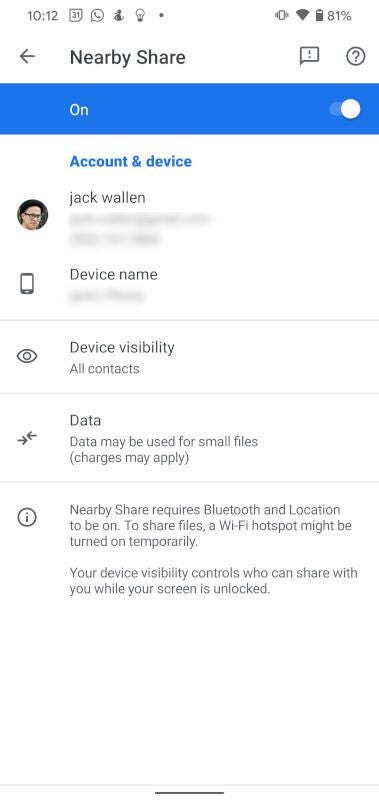In this image, the Nearby Share app is open on a smartphone. The top of the screen displays the title "Nearby Share" flanked by a help icon, an explanation icon, and a back button, all set against a white background. Directly below this, a blue background section indicates that Nearby Share is turned on, with the text reading "ON" and a blue toggle switch positioned to the right.

Further down, the text "Account and Device" appears in blue, signifying different sections within the app. The account associated with Nearby Share is for a user named Jack Wallen, but the detailed information is partially obscured. The "Device name" section reveals the name as "Bled."

In the main body of the screen, the text "Device Visibility: All Contacts" is prominently displayed, accompanied by an eye icon symbolizing visibility settings. Below this, there is a section labeled "Data," which warns that data usage may incur charges if small files are shared, represented by an icon of arrows pointing in opposite directions.

At the bottom of the screen, an information icon with an exclamation inside communicates important details: "Nearby Share requires Bluetooth and location to be on. To share files, hotspots may be turned on temporarily. Your device visibility controls who can share with you while your screen is unlocked." All the text, apart from the highlighted blue sections, is written in black.